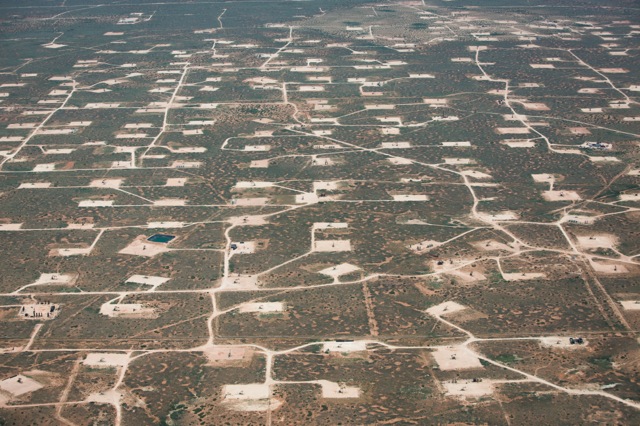The image is an aerial photograph, possibly taken from an aircraft or a satellite, depicting a flat, barren landscape characterized by a repetitive pattern of small, square plots of land. The terrain is a dull brownish-green color, devoid of trees or notable geographical features. Scattered across the landscape are numerous white or light-colored structures, which might be industrial buildings, houses, or possibly part of a farming operation. These structures are interspersed systematically, aligned in neat rows, and each is connected to a network of main roads and smaller roadways that crisscross the area. One prominent road runs diagonally towards the center of the image. The overall scene appears fairly monotonous and lacks vibrant features. While the photo is taken from a high altitude, it is detailed enough that individual cars can still be discerned as they move along the roads.